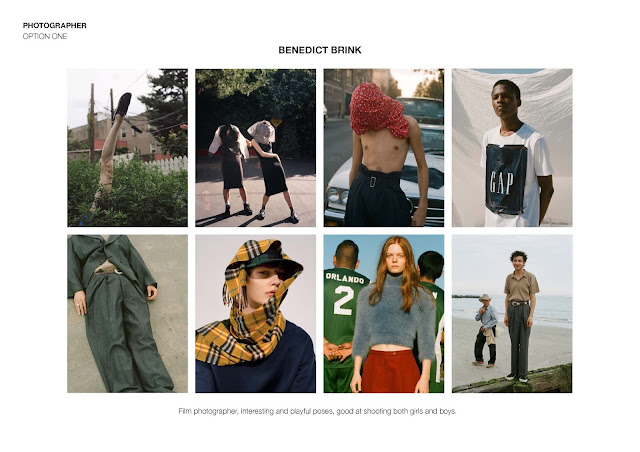The collage features an array of intriguing photographs. At the top, a white background displays the text "Photographer Option 1" and "Benedict Brink" in bold black letters. Below, there are eight distinct images.

- The top left photo captures a foot emerging from a bush. The foot points outward, clad in a black shoe, and reveals a bare leg, knee, and thigh.
- Another photo shows a shirtless man wearing black pants with a silver belt buckle. His face is obscured by a red covering.
- In another image, a Black man stands in front of a white sheet, wearing a T-shirt with the word "Gap" printed on it.
- One photograph features a man staring directly at the camera. He dons a black shirt and a green and blue plaid hat. A yellow, white, and black scarf is wrapped around his head, leaving his face visible.
- Another image depicts the number "2" written on a green shirt.

Each photograph offers a unique composition and subject, collectively creating a compelling visual narrative.